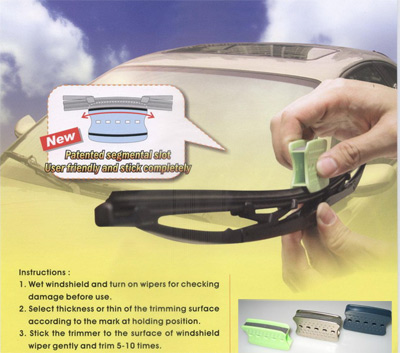The advertisement showcases a product meant for maintaining your windshield wipers. The background features a blue sky with white, puffy clouds framing the corners, and a yellow-tinted car below with a sunroof. Prominently displayed is a man's hands holding a green plastic trimmer against the windshield wiper blade, demonstrating its use. A red tab labeled "new" highlights a speech bubble from the wiper blade, which reads, "Patented segmental slot, user-friendly, and sticks completely."

Instructions occupy the bottom left of the image in black text, outlining three steps: 1) Wet the windshield and activate the wipers to check for damage. 2) Select the thickness of the trimming surface according to the mark on the holding position. 3) Gently stick the trimmer to the windshield wiper surface and trim 5-10 times. 

In the bottom right corner, a gray rectangle features three trimmers in different colors: green, gray, and blue, aligned at an angle. The illustration provides a clear and comprehensive guide for users to maintain and enhance their windshield wipers effectively.